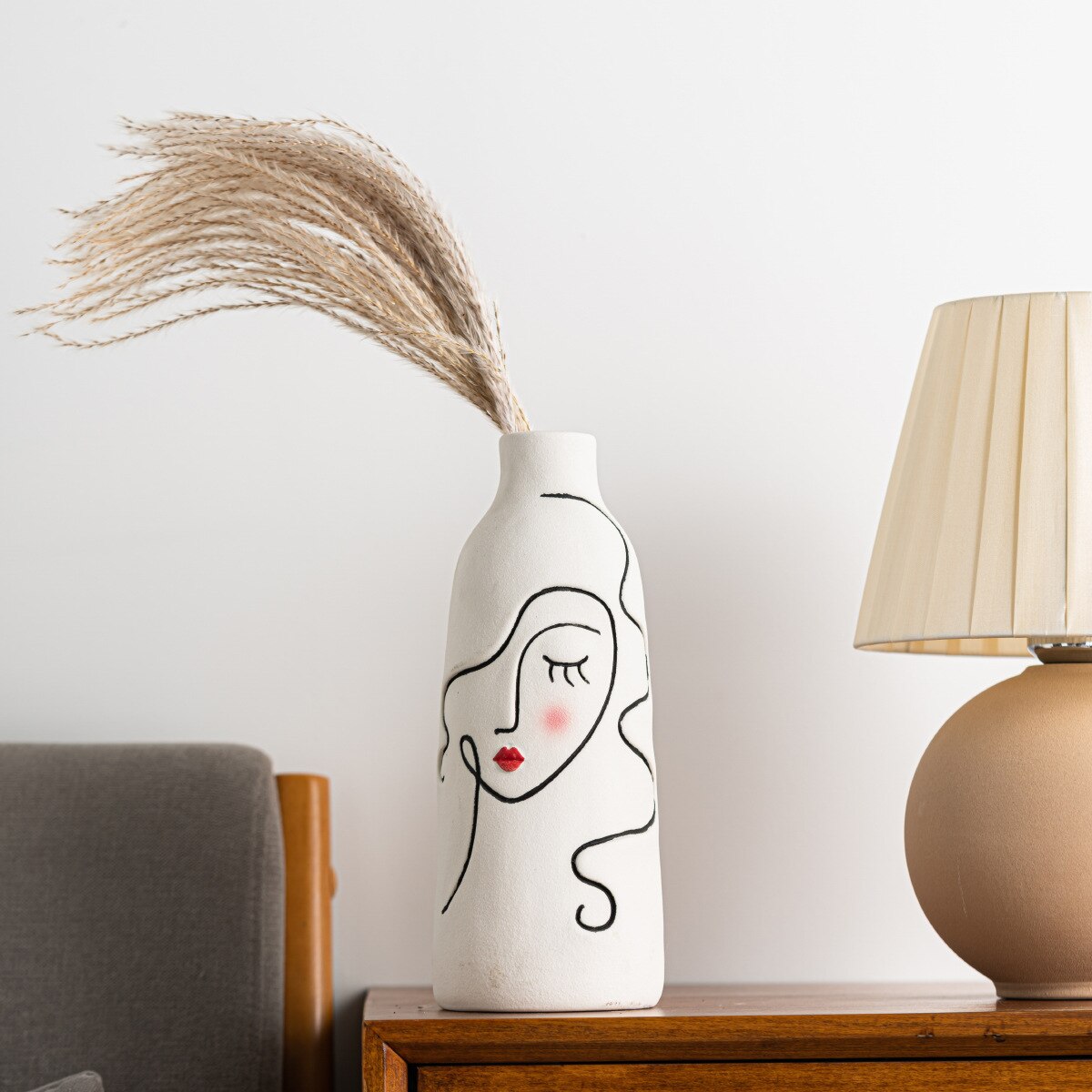The photograph features a quaint living room scene with a white-walled background. Central to the image is a handmade cylindrical vase positioned on a small, brown wooden side table with a drawer. The vase itself is designed with a distinctive tapered shape—wider at the bottom, it narrows slightly towards the top before pinching in at the lip. Predominantly white, the vase features an abstract, artistic rendering of a woman's face. Her facial details are thoughtfully etched with black lines, including a closed eye with three prominent eyelashes, a single-line depiction of her nose and eyebrow, small red lips, and a pink blush spot on her cheek. The woman's hair is represented with fluid, curvy lines, draping over the left side of her face and finishing with a curl at the bottom right. 

From the top of the vase, several strands of tan-colored, fake grass arch slightly to the left. Adjacent to the table, on the right side of the image, is a spherical table lamp with a light brown base and a white, pleated conical lampshade. Completing the scene, a gray couch with wooden trim is partially visible on the left, adding to the cozy ambiance of the room.